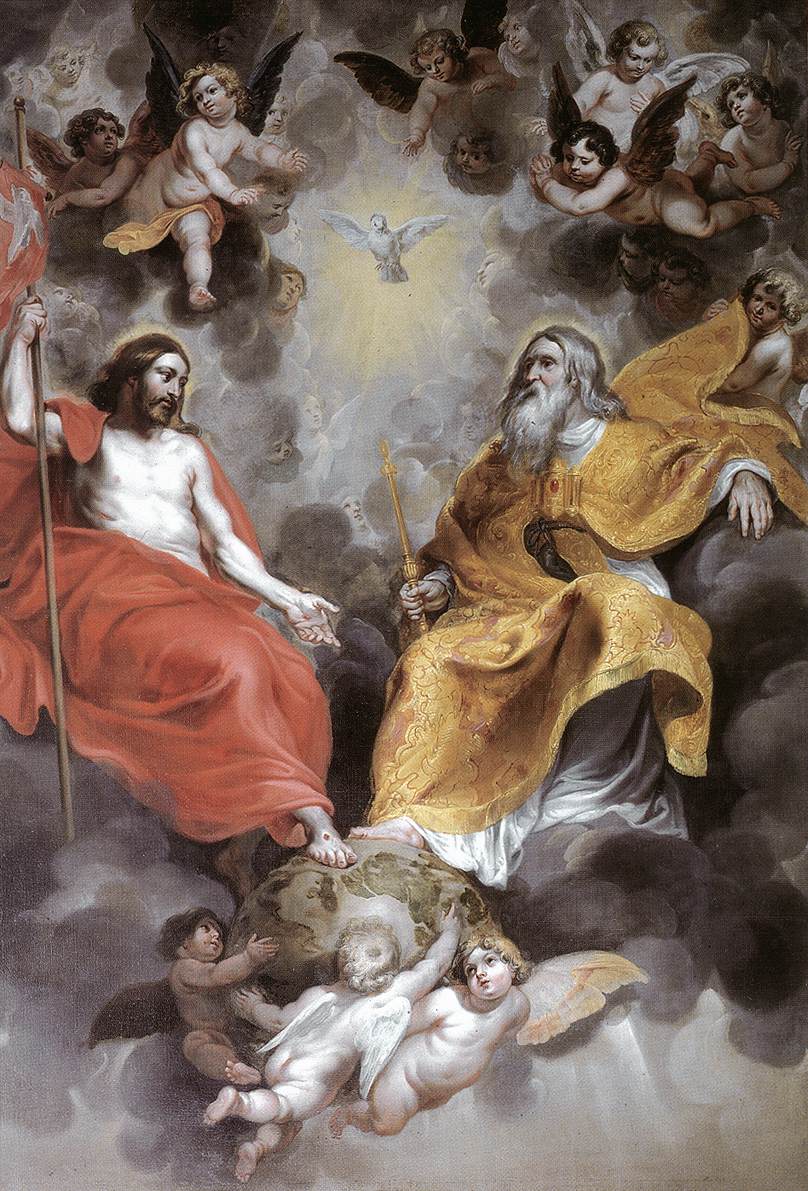The painting appears to be an exquisitely detailed oil painting with a distinct religious theme. At the center, two prominent male figures are seated on dark clouds, surrounded by a multitude of cherubs and angels that are gracefully floating. The figure on the left, who resembles Jesus, is adorned in a flowing red robe that reveals his bare chest and arms. He holds a long staff with a red banner and has a noticeable wound on his foot, which is supported by a rock held by cherubs below. Opposite him, the figure on the right has long silver hair and a beard, and is dressed in an opulent gold cloak over a flowing white undergarment. This figure, possibly representing God, emanates a dignified presence. A radiant white dove, representing the Holy Spirit, takes center stage between the two, adding to the divine aura. The scene is infused with golden light, enhancing the heavenly atmosphere, and the background is filled with soft, billowing clouds and numerous little angels. The entire composition exudes a sense of holiness and celestial grandeur.